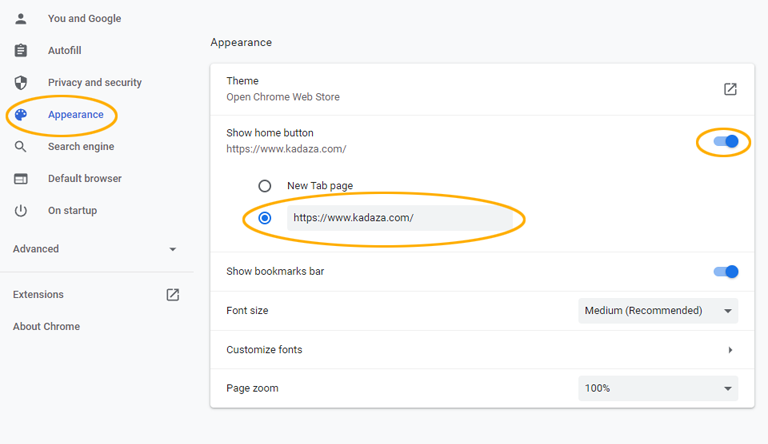This screenshot captures the 'Settings' page within the Google Chrome web browser, showcasing a detailed view of the 'Appearance' settings option. The image itself is a square-shaped screenshot with an off-white background, overlaid by another white square in the center, indicating the active 'Settings' menu.

On the left sidebar, a series of navigational options are listed:
1. You and Google
2. Autofill
3. Privacy and Security
4. Appearance (highlighted)
5. Search Engine
6. Default Browser
7. On Startup
8. Advanced (expandable drop-down menu)

The 'Appearance' tab is highlighted in blue to indicate it is currently selected, and an additional yellow circle emphasizes this selection.

On the right side of the page, within the 'Appearance' settings, further details are displayed. A yellow circle highlights the toggle button in the upper right corner, which controls the visibility of certain appearance settings. Another yellow circle indicates the setting for the 'New Tab' page, which is currently configured to open www.kadaza.com (K-A-D-A-Z-A dot com).

This screenshot provides a comprehensive view of how users can customize their theme and set a custom home page versus using the default settings. The 'New Tab' page configuration specifically shows that it has been changed to kadaza.com, showcasing the flexibility of Chrome's appearance settings.